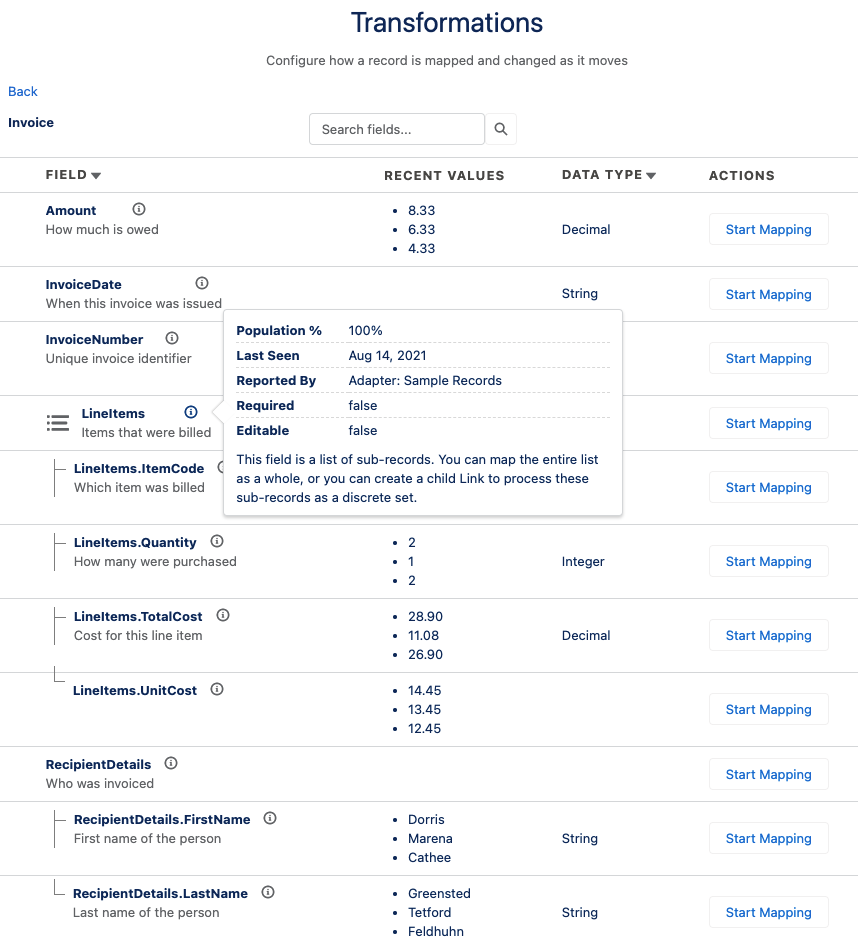This image provides a detailed interface for configuring how records are mapped and adjusted during their processing. At the top of the image, the title "Transformations" is prominently displayed in navy blue font. Below this title, there is a concise description in small black font: "Configure how a record is mapped and changed as it moves."

On the left, in turquoise, the word "Back" is positioned, followed by "Invoice" in navy blue. Just beneath the "Transformations" header, several lines down, is a search box labeled "Search fields" with a magnifying glass icon to its right.

The left-hand column features a menu in all capital letters: "FIELDS" with a down triangle, followed by "RECENT VALUES," "DATA TYPE" with another down triangle, and finally "ACTIONS." Within the fields column, various entries are listed. 

- **Amount** (navy blue) with a description "How much is owed" (black). An information icon (a lowercase 'i' in a circle) is present next to each navy blue entry.
- **Invoice Date** (navy blue) with the description "When was this invoice issued?" (black).
- **Invoice Number** (navy blue) with "Unique invoice identifier" (black).
- **Line Items** (navy blue, one word) with the description "Items that were billed" (black). 
- **Line Items.Item Code** (navy blue) under "Line Items," described as "Which item was billed" (black).

Following this, more line item details include: **Line Items.Quantity** ("How many were purchased"), **Line Items.Total Cost** ("Cost for this line item"), and **Line Items Unit Cost**.

A pop-up overlay next to the "Line Items" has a white background. It lists:

- **Population Percentage** (navy blue) followed by "100 percent" (not bold).
- **Last Seen** (bold, navy blue) followed by "August 14, 2021" (not bold).
- **Reported By** (bold, navy blue) followed by "Adapter: Sample Records" (not bold).
- **Required** (bold) with "False" on the right (not bold).
- **Editable** (bold) with "False" on the right (not bold), and a note stating, "This field is a list of sub-records. You can map the entire list as a whole, or you can create a child link to process the sub-records as a discrete set."

Continuing in the main column:
- **Recipient Details** (bold, navy blue), with "Who was invoiced" (black).
- **Recipient Details.First Name** with "First name of the person" (black).
- **Recipient Details.Last Name** with "Last name of the person" (black).

Under the "Recent Values" and "Data Type" columns, actual data and types are listed but partially obscured by the pop-up. The "Actions" column shows "Start Mapping" in turquoise next to each field.